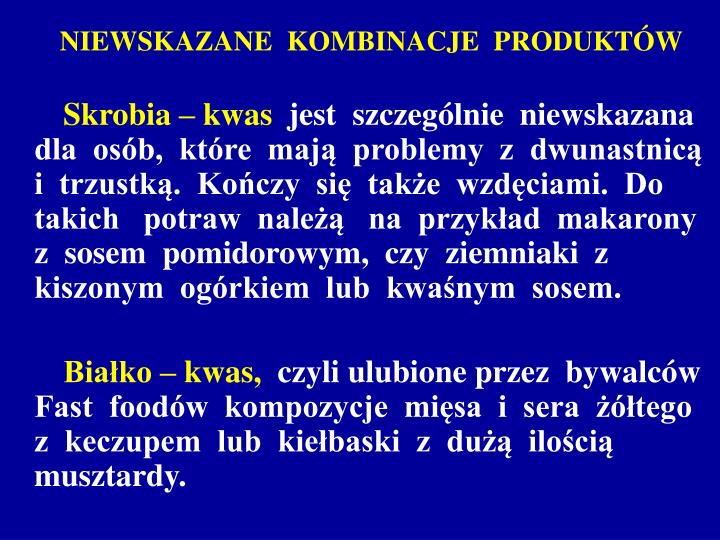The image is a horizontally-oriented color infographic with a dark medium blue background. It features a prominent headline in a yellow serif all-cap font written in Polish, positioned at the top. Below the headline, there are two distinctly formatted paragraphs. The first paragraph, consisting of six lines of white text, begins with an introductory line in yellow text and is aligned to the left with the first line indented. Similar formatting is followed in the second paragraph, which contains four lines of white text, preceded by another line of yellow introductory text. Both paragraphs begin with a few words in yellow, emphasizing key points. The infographic combines visual and textual elements, and appears to relate to production, given the partial translation of a few words.